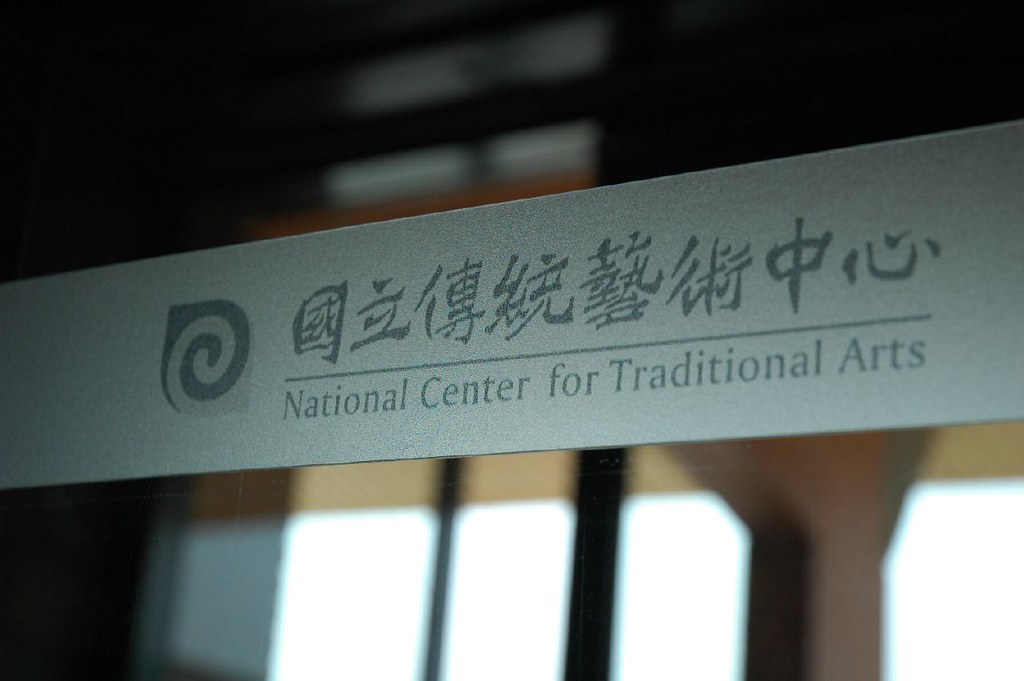The image depicts a slightly tilted wide rectangular sign indoors, set against a background featuring tall, black-bordered windows partially covered by beige shades at the top, with the rest of the scene being blurry and dark, giving a shadowy appearance. The sign, which is a grayish light green color, starts near the top right and extends diagonally downward. On the left side of the sign, there is a distinctive dark green swirly symbol resembling a lemon shape with a pointy corner. To its right, eight Chinese characters are written in dark green and underlined. Beneath the characters, the phrase "National Center for Traditional Arts" is inscribed in the same dark green color, with each word capitalized except for "for." The sign appears to be in front of an office or center.